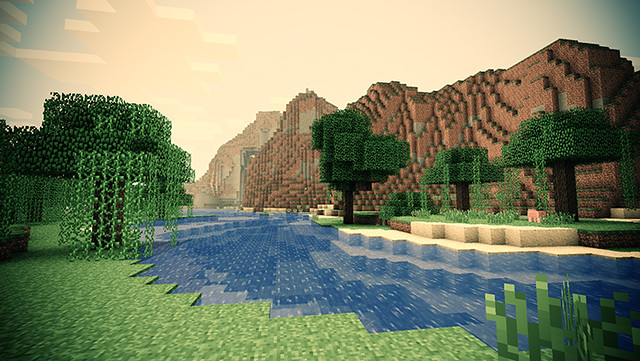This computer-generated rendering vividly depicts a serene river scene teeming with natural elements. At the heart of the composition is a meandering river that originates from the lower right corner, weaving its way through the center before veering left and continuing into the background. The river's water is a striking shade of blue, juxtaposed against lush greenery that flanks its banks. To the right of the river, three to four trees are artfully arranged in a landscaped area, offering a sense of depth and organization. Meanwhile, to the left, a couple of large trees stand proudly, adding balance and contrast to the scene. In the distance, majestic mountains border the horizon, providing a grand backdrop that frames the entire setting. The characters within the scene are uniquely square-shaped or composed of wiggly lines that approximate square forms, lending a distinctive, almost whimsical quality to the artwork. This rendering masterfully combines detailed natural elements with creative, geometric characters to create a harmonious and enchanting landscape.